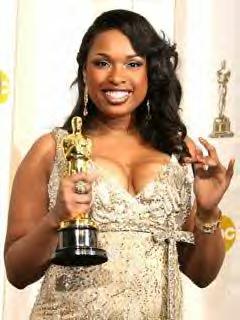The image features a close-up of Jennifer Hudson, showcasing her radiant smile and elegant appearance. She has long, black hair parted to the side, and she is wearing eye-catching dangle earrings. Her sparkling gold dress, featuring thin straps, adds to her glamorous look. Jennifer is holding a golden Grammy award with one hand, while her fingers of the other hand are gracefully displayed, palm facing outwards. The background consists of a mostly white curtain, creating a light backdrop that highlights Jennifer and the metallic award prominently. Additionally, a second golden Grammy award is visible on a pedestal behind her, and there is an ABC symbol near the lower right-hand corner of the image. The photo is vertically oriented in the shape of a rectangle.